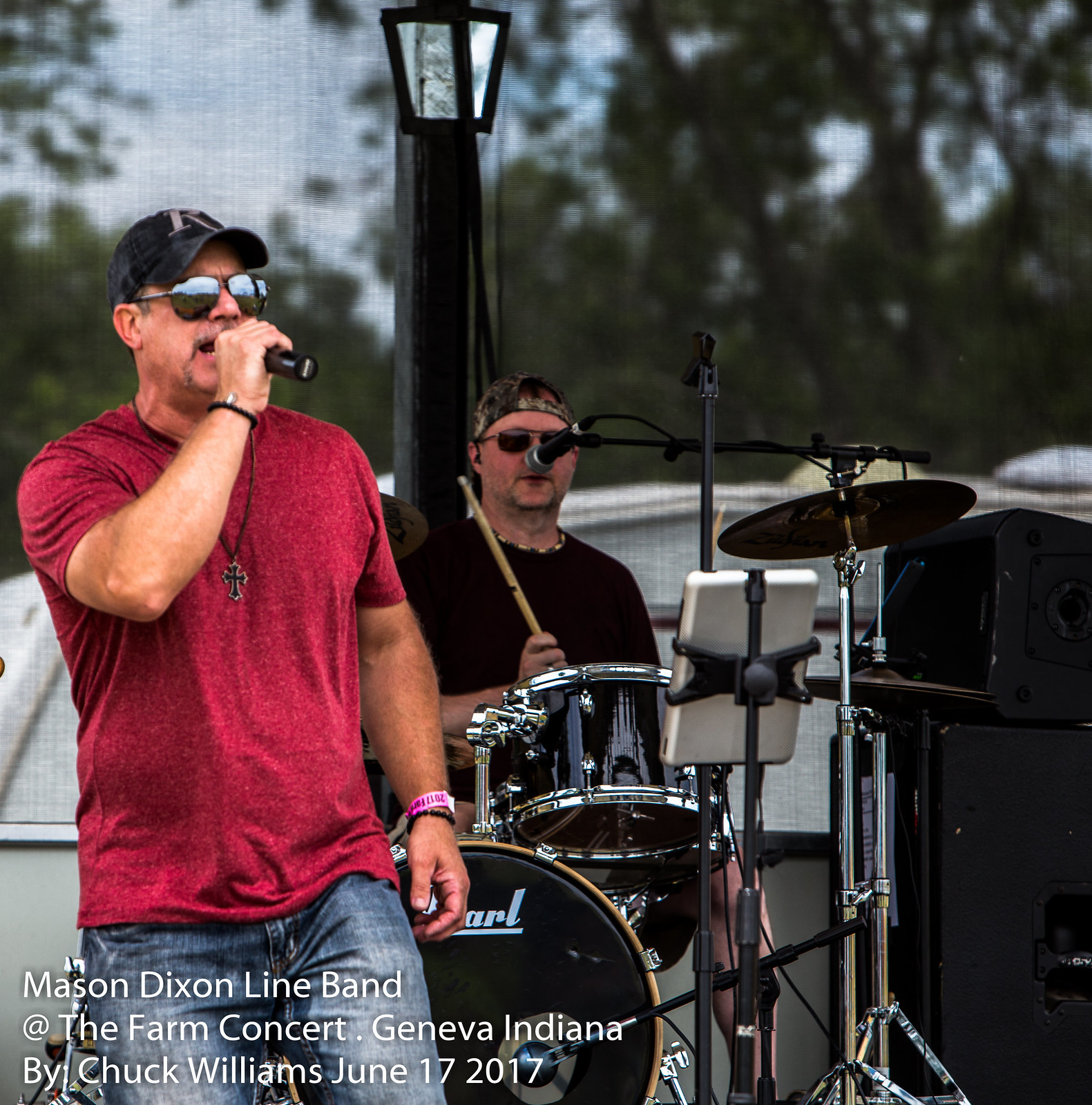The image captures an energetic performance of the Mason Dixon Line Band at the Farm Concert in Geneva, Indiana, held on June 17th, 2017. On the left, a man, clad in a red T-shirt and blue jeans, accessorized with a black cross necklace, mirrored sunglasses, and a blue ball cap featuring a letter 'R', passionately sings into a microphone. An iPad mounted on a stand in front of him likely serves as a lyrics prompt. To his right, the drummer, also wearing sunglasses and a backwards cap, plays behind an extensive black drum set. He is seen gripping a drumstick, his black T-shirt contrasting with the sky and trees visible through a scrim in the blurry background. A lamppost and a faint outline of a white vehicle add subtle details to the outdoor setting. The caption in the lower left corner, written in white ink, reads: "Mason Dixon Line Band at the Farm Concert Geneva, Indiana by Chuck Williams, June 17th, 2017."